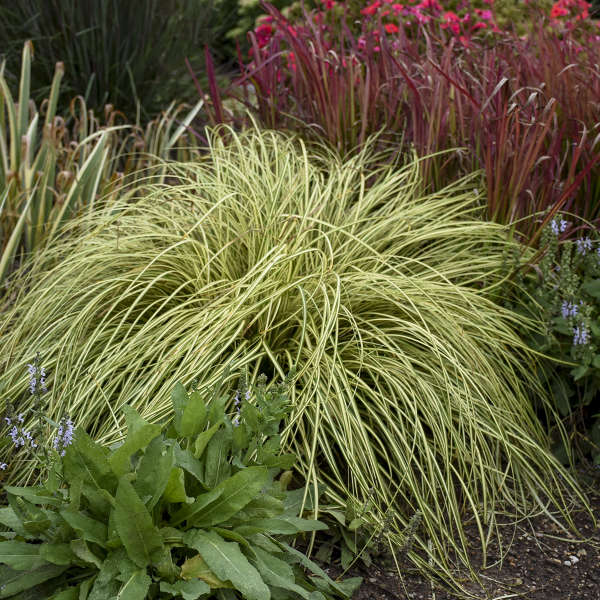This outdoor photograph showcases a diverse array of flora, likely positioned in a controlled or botanical environment. Dominating the center is a large ornamental grass with blades arching outward, exhibiting a light green hue. Flanking this centerpiece on the left, there is a plant resembling crabgrass, marked by its bushy appearance and verdant color. Directly in front of the ornamental grass, a vibrant green weed stands prominently. Moving to the right, the scene transitions into a captivating display of tall stalks with striking reddish-pink flowers at their tops. Meanwhile, interspersed among the foliage are stems with periwinkle petals, contributing a splash of delicate color. At the base of this plant ensemble, the ground is bare dirt, suggesting a deliberate planting in an organized setting. The top left of the photograph hints at additional green foliage, adding to the lushness of the scene. This detailed composition of varying plant life, from grasses to colorful blossoms, creates a rich tapestry of texture and color.